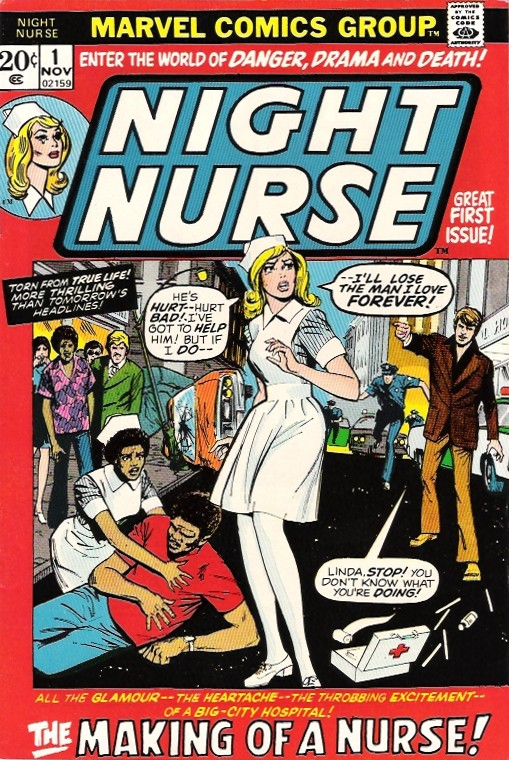This scan captures the cover of a vintage Marvel comic book titled "Night Nurse." The cover features a striking red background with a bold black band across the top. Within this band, in large yellow letters, it reads "Marvel Comics Group," and to the left, "Night Nurse" is written in lighter text. Below this band, the price "20¢" appears in a white box, along with the issue date "November 1" and the code "02159."

Centered prominently, a blue box with a black outline displays the title "Night Nurse" in large white letters. Below the title, a dramatic scene unfolds in the middle of a street. A nurse, identified as Linda, stands with a shocked expression, her blonde hair flowing to her shoulders, and a speech bubble saying, "He's hurt hurt bad... I've got to help him but if I do, I'll lose the man I love forever." Kneeling nearby is another nurse tending to a wounded man lying on the ground, holding his side. Scattered first aid materials and an open kit lie on the pavement.

To the right of Linda, a man in a brown suit points at her, exclaiming, "Linda, stop! You don't know what you’re doing." In the backdrop, a police officer is seen running toward the chaotic scene, adding to the sense of urgency. Further back, bystanders and an overturned car hint at a recent traumatic event.

Across the top, the tagline in white letters reads, "Enter the world of danger, drama, and death," setting the tone for the comic’s thrilling content. At the bottom, in smaller yellow text, it proclaims, "Torn from true life, more thrilling than tomorrow's headlines." Right beneath this, in larger white letters, it announces, "The making of a nurse. Great first issue!" capturing the essence of the comic's dramatic and suspenseful narrative.